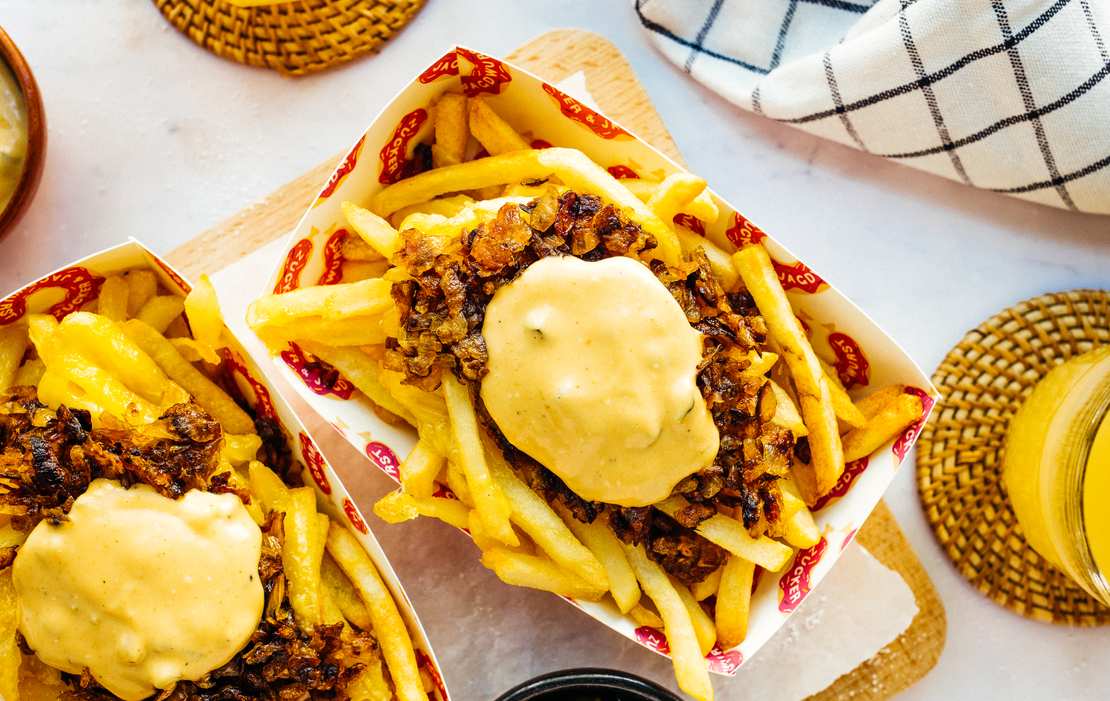The image depicts a table set with a variety of items, including cups filled with what appears to be orange juice and a dish towel. At the center, two paper boats branded with a logo, positioned side by side, hold crispy, thin French fries. These fries are generously topped with finely browned, grated meat that resembles sautéed onions or bacon. Atop the meat, a scoop of a gooey, cheesy mixture sits, which has a pinkish hue and specks of something green, possibly jalapenos or pickles. The scene is rich with textures and colors, offering a visually appealing arrangement of delicious food and drink.